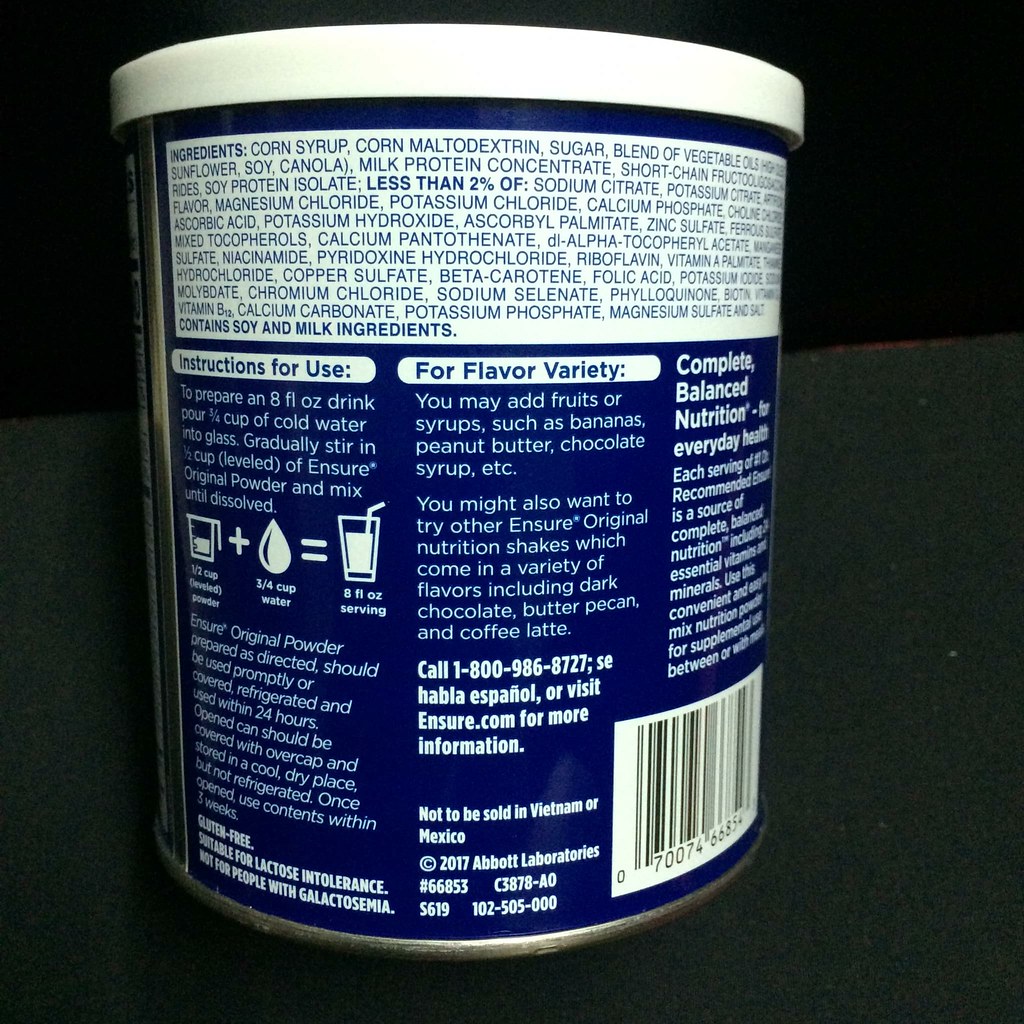A close-up image of an Ensure Original Powder container displays its detailed label. The label lists the product's ingredients and provides instructions for use, which include preparing an 8 oz drink by gradually stirring in ½ cup of Ensure Original Powder into 3 quarts of cold water in a glass, and mixing until dissolved. The product is suggested for improving bone health among other benefits. The label also mentions the flavor variety options, encouraging users to enhance the drink's taste by adding fruit or other ingredients. Additionally, the label includes a bar code and the text "2017 Abbott Laboratories," indicating the manufacturer, and highlights that the product is gluten-free and offers complete balanced nutrition for everyday health. The container features a white lid, a clean white backdrop for the ingredient information, and a blue section at the bottom with additional product details.